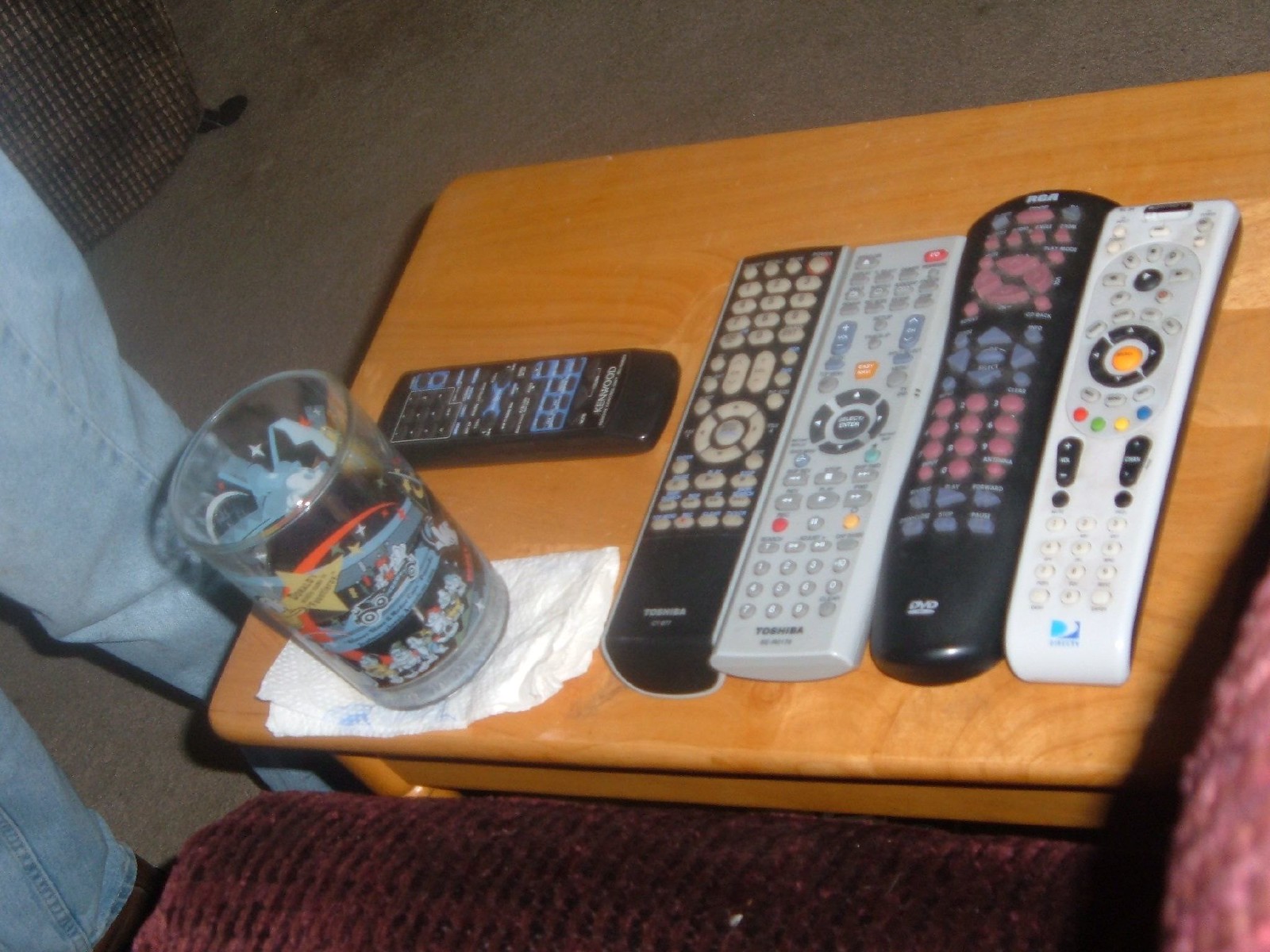The image captures a cluttered wooden coffee table, set in a dimly lit living room with dark brown carpeting. The table is a medium to light-colored wood and hosts an array of items. On the left-hand side of the table, resting on a folded white napkin, is a glass adorned with colorful, intricate designs, including Disney characters such as Mickey Mouse in a Fantasia hat and possibly the Seven Dwarfs. The glass is positioned near the bottom left corner.

Above the glass, a small remote control, black with blue trim, lies horizontally. Beyond this, four larger remote controls are arranged vertically in a row, each distinct in appearance. The first remote on the left is black with gray buttons, the next is mostly gray with several blue and red buttons scattered throughout, another remote is long and black with predominantly red and blue buttons, and the final remote is white with a circular black center and a distinctive yellow button, accompanied by red, green, yellow, and blue multi-function buttons at the bottom.

Partially visible near the table's edge, a person in blue jeans stands, their legs casually posed as they oversee the scene. The ambient room includes hints of furniture upholstered in burgundy fabric and a cushion in the background, contributing to the cozy yet retro atmosphere dominated by older, bulky electronics.